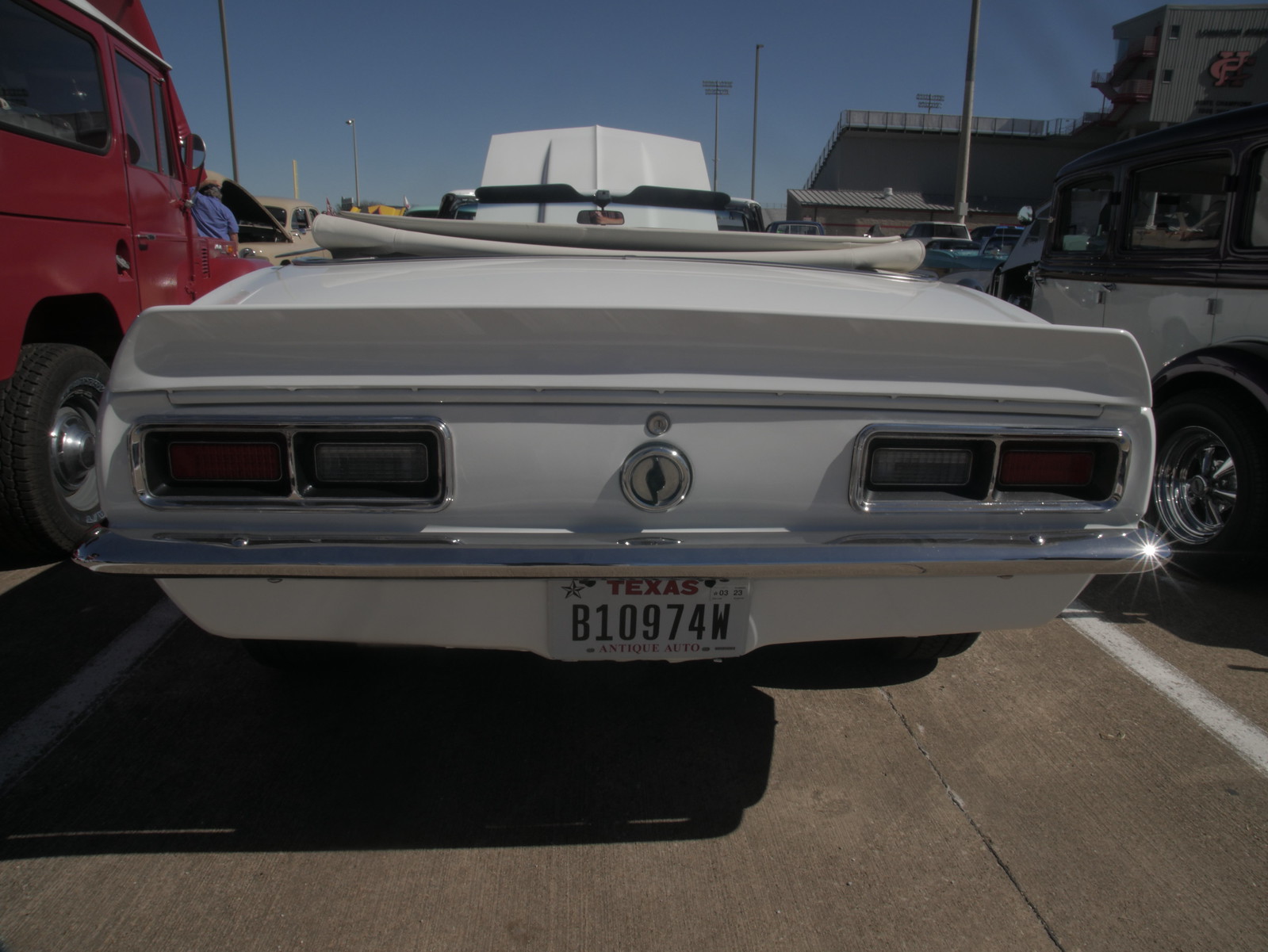This image captures a close-up view of the rear of a classic white convertible, possibly from the 1960s or 70s, highlighting its retro design. The car's taillights are visible on both the left and right, accompanied by a trunk keyhole with a mysterious round silver area below it. The vehicle's license plate reads "Texas B10974W." The convertible’s top is folded back, and part of the windshield and rearview mirror is visible. The hood of the car is open, suggesting it might be on display. The car is parked on a black asphalt surface with white parking lines, indicating it’s in a parking lot, likely at a car show. To the left, a red truck and, to the right, a classic white and black hot rod are parked. In the background, there are structures that appear to be part of a stadium, and various buildings with gray roofs and tan siding. The setting is lit by multiple light posts, and the image was taken during the daytime.